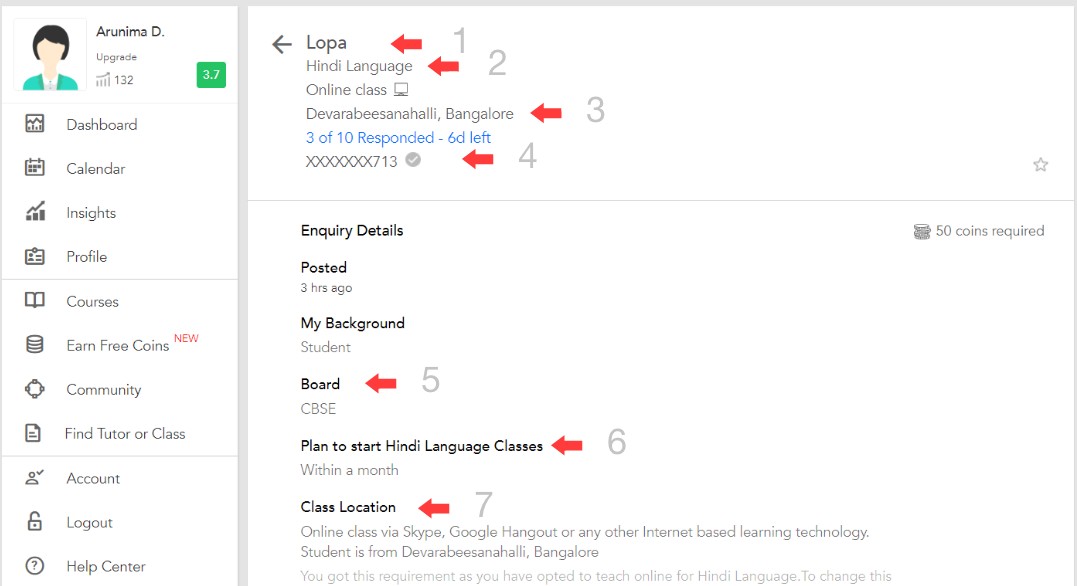In the depicted image of a web page, the layout is composed of a sidebar on the left and a larger main display to the right. The sidebar serves as a navigation menu with a user profile section at the top. The profile section includes a cartoon image of a person next to the name "Arunama D," indicating the user's identity.

Below the profile, the sidebar features a vertical list of navigation buttons, each leading to different sections or functionalities. The options are listed as follows, from top to bottom: Dashboard, Calendar, Insights, Profile, Courses, Earn Free Coins, Community, Find Tutor or Class, Account, Logout, and Help Center.

On the main section of the web page, the topmost element is a label reading "Lopa," accompanied by an arrow pointing to the left. Directly beneath this label, there's a heading that reads "Handy Language, Online Class, Devara, Bisana, Hali, Bangalore," followed by a note indicating "Three of ten responded."

Further down in the main content area, there are several categorized sections: "Inquiry Details," "Posted," "My Background," "Board," "Plan to Start Handy Language Class," and "Class Location." These sections likely contain detailed information relevant to the user's language class inquiries and planning.